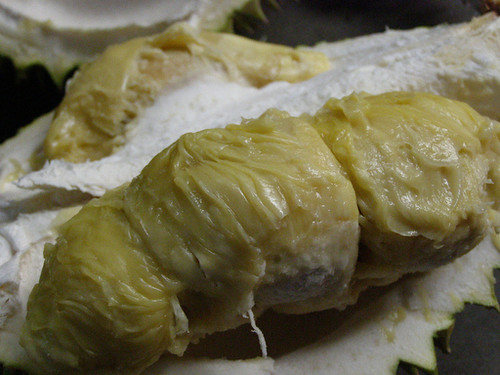This close-up color photograph captures the interior of a durian fruit, revealing its unique and distinctive details. In the center of the image, there are three equal segments of the durian's yellow, custard-like flesh, which appears wrinkled and buttery, suggesting a rich, creamy texture possibly coated with congealed fat or a sticky glaze that developed after cooking. These segments are resting on a surface that could be pastry dough or the shell of the fruit. To the front of the durian, there is a sprinkling of white powder, likely flour. In the background, another instance of the durian fruit can be seen, and the setting features a black cloth that the food is laid upon.